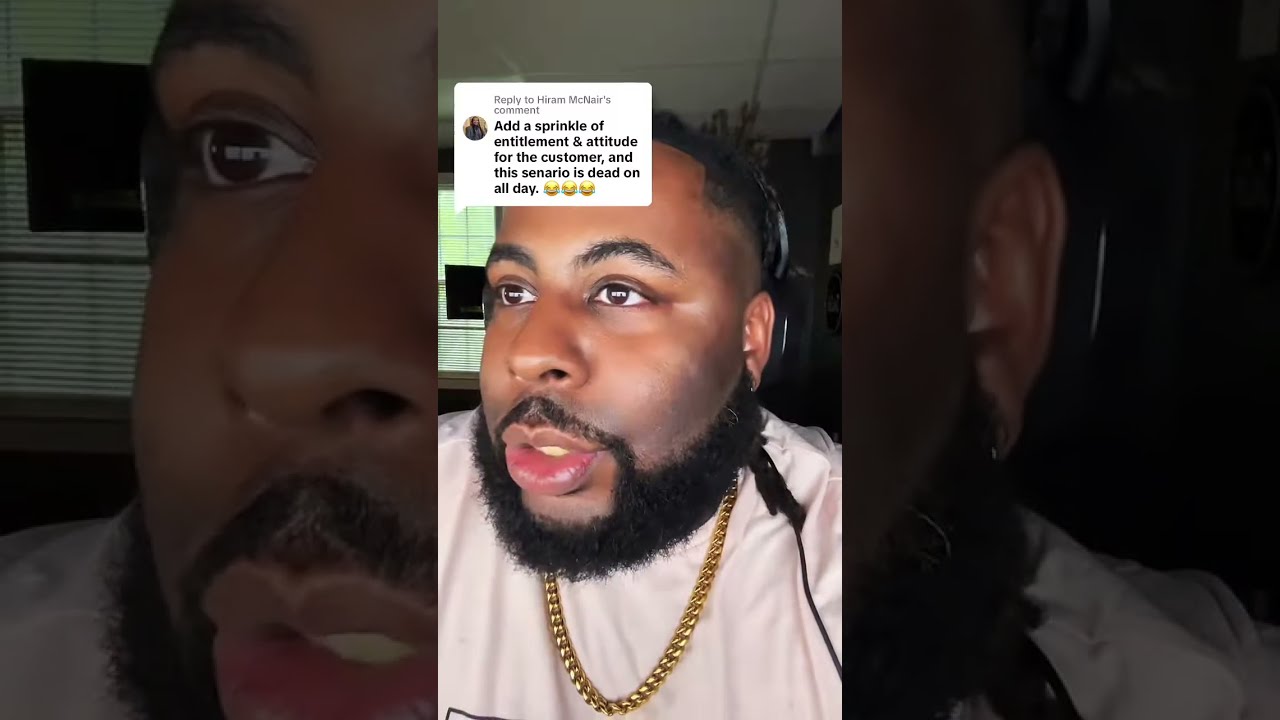The image features a young black man with dark skin, a full beard, and dark eyebrows, wearing a white shirt and a gold chain around his neck. He is looking towards the left, with his lips pursed together and a contemplative expression. He has headphones on, with a black cable visible along the right side of his shoulder. The background shows a window and a ceiling with a light green tint, indicating that he is indoors and alone. The image is sharply focused on his face, while the zoomed-in columns on the left and right are more tinted. Above his forehead, there is a white box containing black text that reads, "Add a sprinkle of entitlement and attitude, and the customer in this scenario is dead-on all day," followed by three laughing emojis, and it is a reply to Hiram McNair's comment.